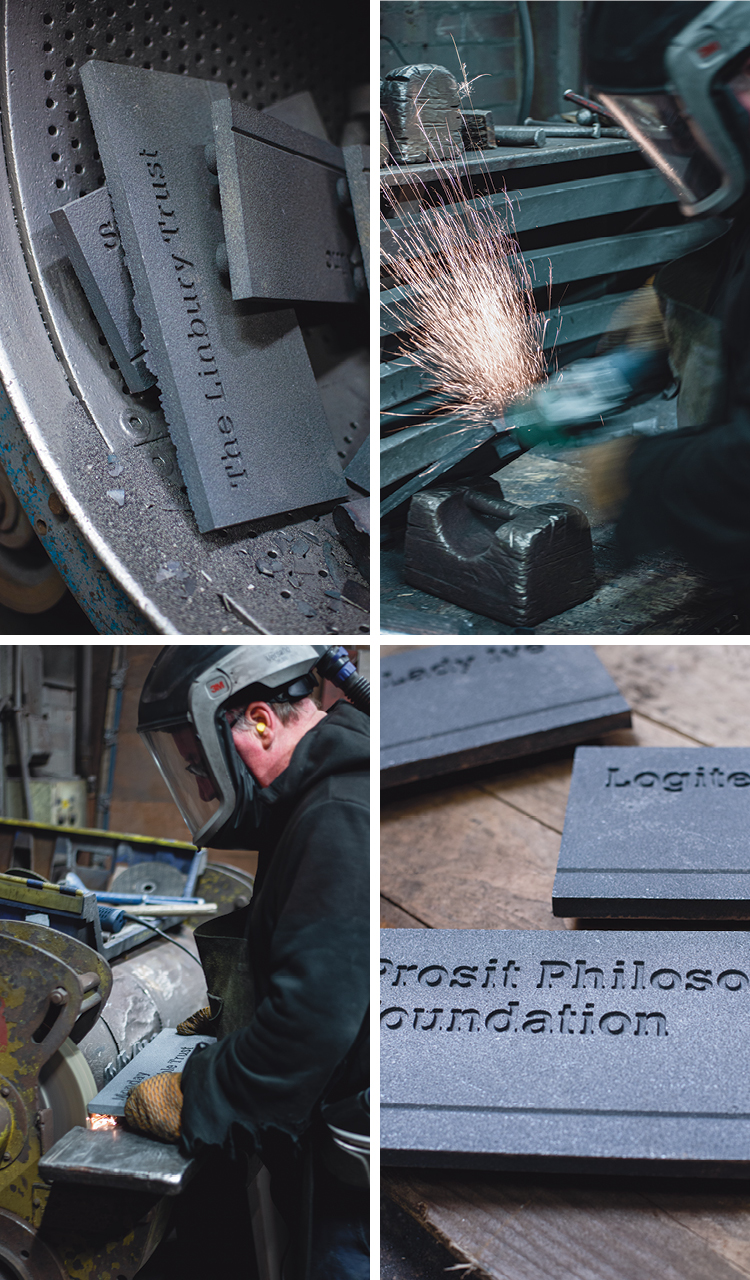The image is composed of four vertically oriented photographs arranged in a two-by-two grid, depicting a detailed view of a bustling metal shop where workers are crafting and engraving metal plates. In the top left photograph, slabs of metal, possibly granite, feature etched text such as "The Linbury Trust." Directly to the right, in the top right quadrant, a worker, dressed in protective gear and a welding helmet, is seen cutting metal with a tool, causing sparks to fly as he works. This dynamic scene captures the intensity and precision of his craft. The bottom left image similarly features another worker at a workbench, actively fabricating or smoothing out a metal plate with intricate text. The final bottom right photograph shows a collection of these engraved metal plates with assorted writings, laid out on a table within the workshop environment. Overall, the images collectively showcase the process and skill involved in creating personalized plaques or signs within a metal shop, capturing both the human element and the finished products.